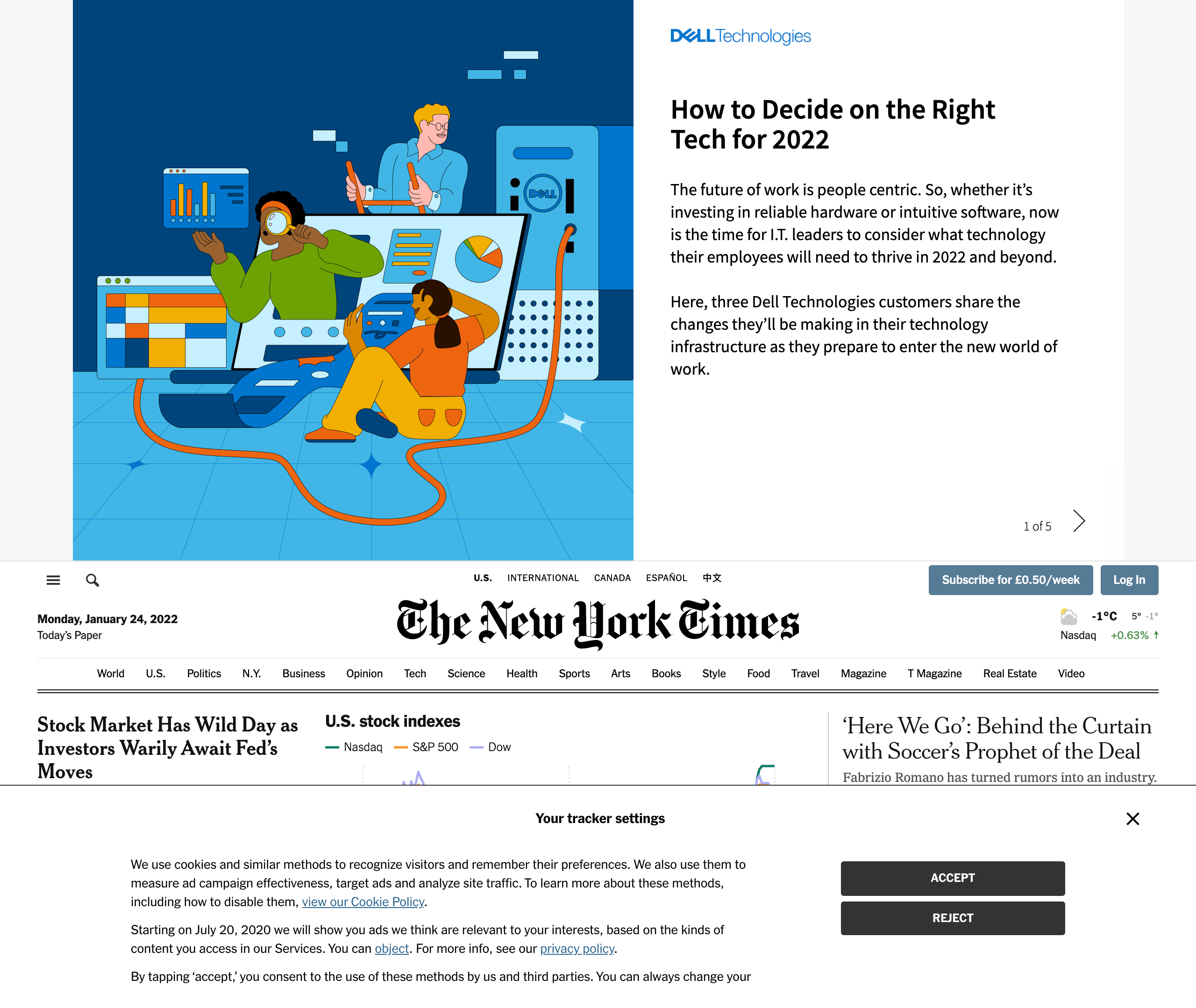The image appears to be a composite of two separate images stacked one above the other.

In the bottom image, set against a white background, the prominent text reads "The New York Times" in bold black letters. Above this title, there is a smaller font featuring the links "U.S.," "International," "Canada," "Español," and some Asian characters. The "U.S." link is in bold, suggesting that it's the currently selected section. Below this level, there’s a category menu listing various sections such as "World," "U.S.," "Politics," "New York (NY)," "Business," "Opinion," "Tech," "Science," "Health," "Sports," "Arts," "Books," "Style," "Food," "Travel," "Magazine," "T-Magazine," "Real Estate," "Video." 

Directly underneath the categories is a headline in black text: "Stock market has wild day as investors warily await Fed's moves." Following this, there is information on U.S. stock indexes, with NASDAQ and S&P 500 mentioned as being down. The text continues to elaborate on coverage titled "Behind the Curtain," revolving around soccer's profitability and mentioning Fabrizio Romano, a figure credited with turning transfer rumors into an industry standard.

A pop-up notification reads, "Your tracker settings," which discusses cookie usage and tracking consent with options for acceptance or rejection. 

The top image has a white background with text related to Dell Technologies. In black text, it reads "How to Decide on the Right Tech for 2022." On the left side of this section, there is an image predominantly featuring shades of blue. This illustration seems to depict several individuals: one person examining charts, another person on a ladder, and a third person engaged with electronic equipment.

This detailed composite captures a snapshot of New York Times website elements and an advertisement for Dell Technologies.